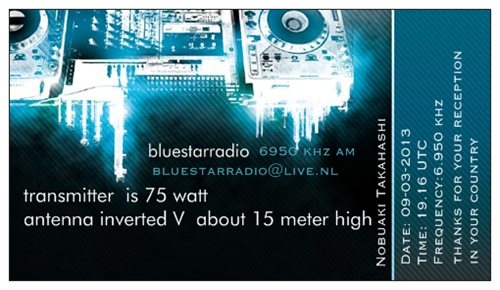The image presents a small rectangular business card with a predominantly blue background accented in white and black. Dominating the left side of the card, the title "Blue Star Radio" is prominently displayed, with an upside-down image of a boombox subtly integrated into the background. Centered below the headline, technical details are provided in white text, stating, "Transmitter: 75 watt, Antenna: Inverted V, about 15 meters high." On the right-hand side, oriented vertically, additional information is listed: "Date: 9-3-2013, Time: 19:16 UTC, Frequency: 6950 kHz AM." A note of appreciation at the bottom right reads, "Thanks for your reception in your country," underlining the card’s purpose related to radio broadcast reception. The recipient's email "BlueStarRadio@Live.nl" is also indicated on the card. Overall, the card appears to serve as a detailed technical and contact information sheet for Blue Star Radio.